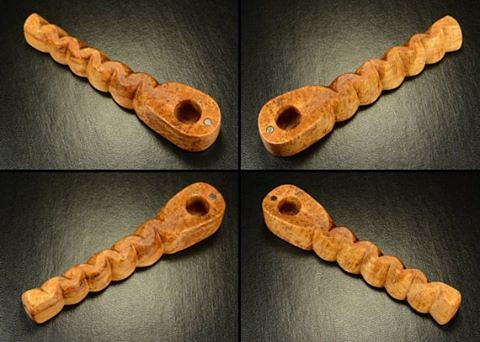The image features a composite arrangement of four slightly varied photographs of a single, hand-carved wooden pipe. Set against a black background with centered, illuminated white spots indicating light sources, each rectangular section of the composite positions the pipe at different angles, creating an X shape with their bowls converging at the center. The wooden pipes, mid-tone brown and intricately carved, resemble small smoking pipes with oval-shaped bowls and wavy stems, akin to small hash pipes. Each pipe has a small bolt-like feature at the top, reinforcing their crafted detail. The distinct arrangement and lighting variation give the whole composite a dynamic symmetry, enhanced by a white cross that runs through the middle, separating the four images.